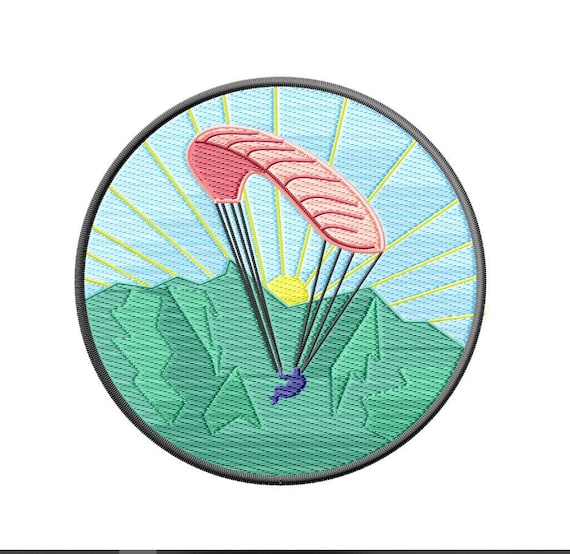The image features a circular patch bordered in black. Inside the patch, a jagged green mountain dominates the center, capped by a yellow sun nestled between two of its peaks. Rays of sunlight radiate from the sun's center in vivid yellow lines. Hovering above the mountain is a pink, hot dog-shaped parachute adorned with horizontal stripes. From the parachute, four black strings on each side descend to a small purple figure, representing a person parachuting through the air. Below the patch, outside the circular boundary, is a distinct black line.